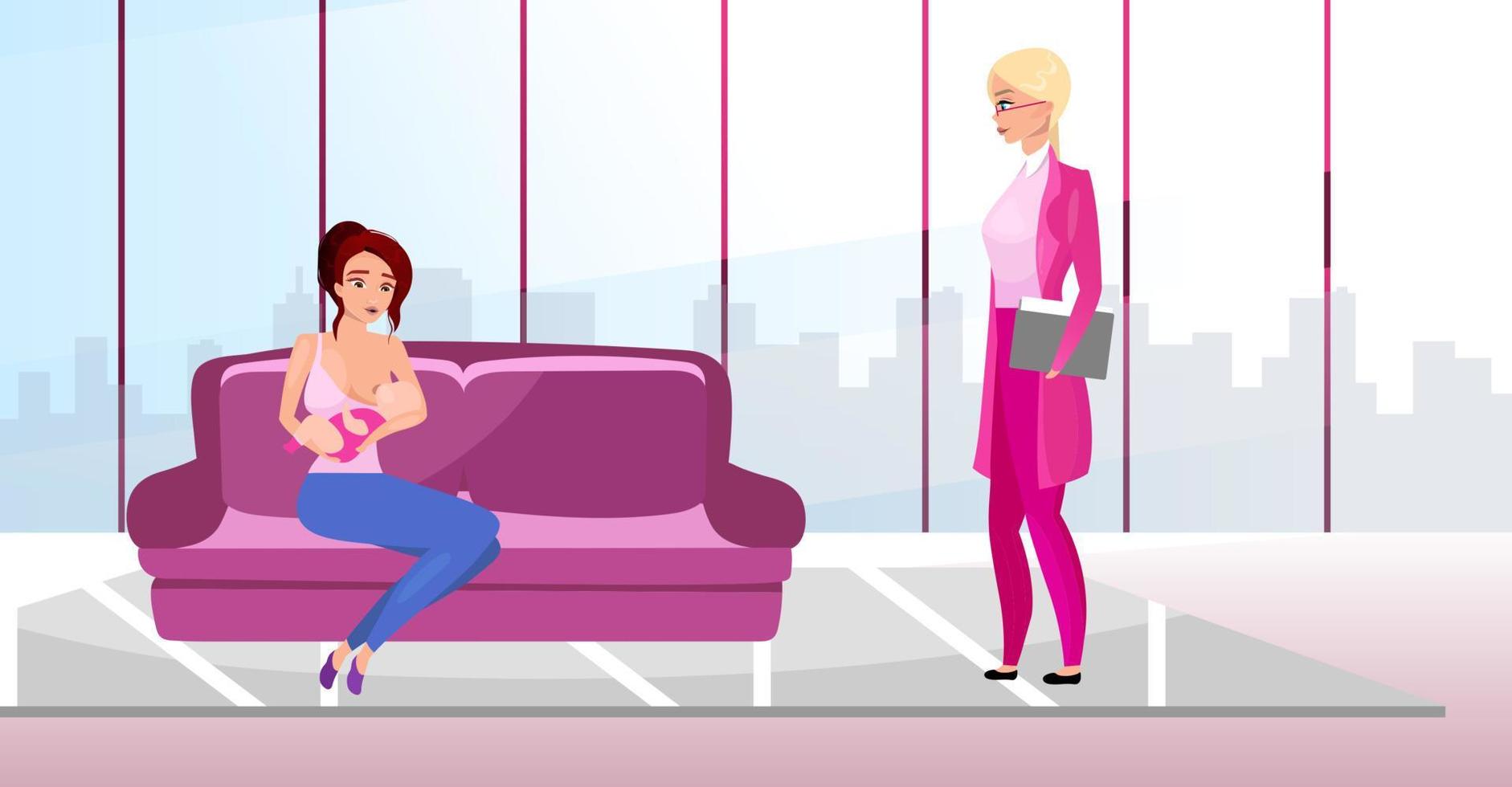This is a highly detailed digital illustration depicting two cartoon women in an upscale city apartment, emphasized by floor-to-ceiling glass windows that reveal the cityscape behind them. The surface beneath them appears to be a clear pane of glass over a cream-colored carpet. To the left, a woman with dark brown hair, potentially wearing a black hat, sits on a pink couch breastfeeding her baby. She is dressed in blue jeans and a pink tank top with purple shoes. Her breast and part of her nipple are exposed to allow the baby to nurse. To the right, another woman, who has blonde hair and wears glasses, stands looking at the seated woman as though they are engaged in a conversation. She is dressed in a pink pantsuit with a lighter pink top and a white collar, and she is holding a folder or book. The scene subtly suggests a commentary on the differing roles of women in society, particularly contrasting the professional workplace with motherhood.